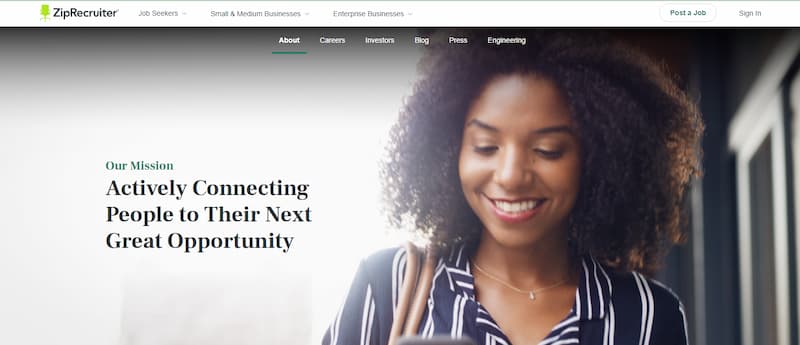The image features a professional setting with a detailed background and foreground elements. On the left-hand side of the image, there is a lime green chair. To the right of the chair, a banner or digital display shows the words "ZipRecruiter" in black font, alongside "Job Seekers." Below this, the options "Post a Job" and "Sign In" are visible. 

The background has a gradient transition starting from dark gray at the top, fading to white in the center, and returning to gray at the bottom. On the right side of the image, through what appears to be a window, a person can be seen.

The person in the image has brown skin and curly hair, and she is wearing a brown necklace. A beige strap is visible on her left shoulder, suggesting she is carrying a bag. She is wearing a blue and white shirt, smiling with red lipstick, and looking down. Above her head, there is white text displaying a list of words in green: "Careers, Investors, Blog, Press, Engineering." On the left side in green text, it reads "Our Mission." The text in black following this reads: "Actively Connecting People to Their Next Great Opportunity," with each major word capitalized for emphasis.

Overall, the composition of the image combines marketing elements with a professional and inviting tone, indicating a focus on career opportunities and connectivity.